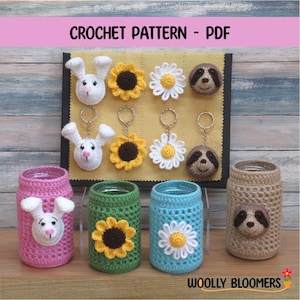This photograph showcases an exquisite display of handmade crocheted products against a cozy wooden wall backdrop. At the top of the image, against a pink rectangle, the words "Crochet Pattern - PDF" are prominently visible, indicating the products are available as downloadable patterns. Hung neatly on a mat, the display features approximately eight beautifully crafted items, including intricate designs of a white rabbit, a vibrant sunflower, a delicate white flower resembling a daisy, a whimsical crocheted button, and what appears to be an adorable sloth. Beneath this selection, a row of four charming cozies or containers for canned drinks is arranged on the table, echoing the same delightful designs. In the lower right corner, the watermark and logo of the business, Wooly Bloomers, subtly mark the image, adding an authentic touch. The overall composition exudes creativity and warmth, highlighting the detailed craftsmanship of each crocheted piece.